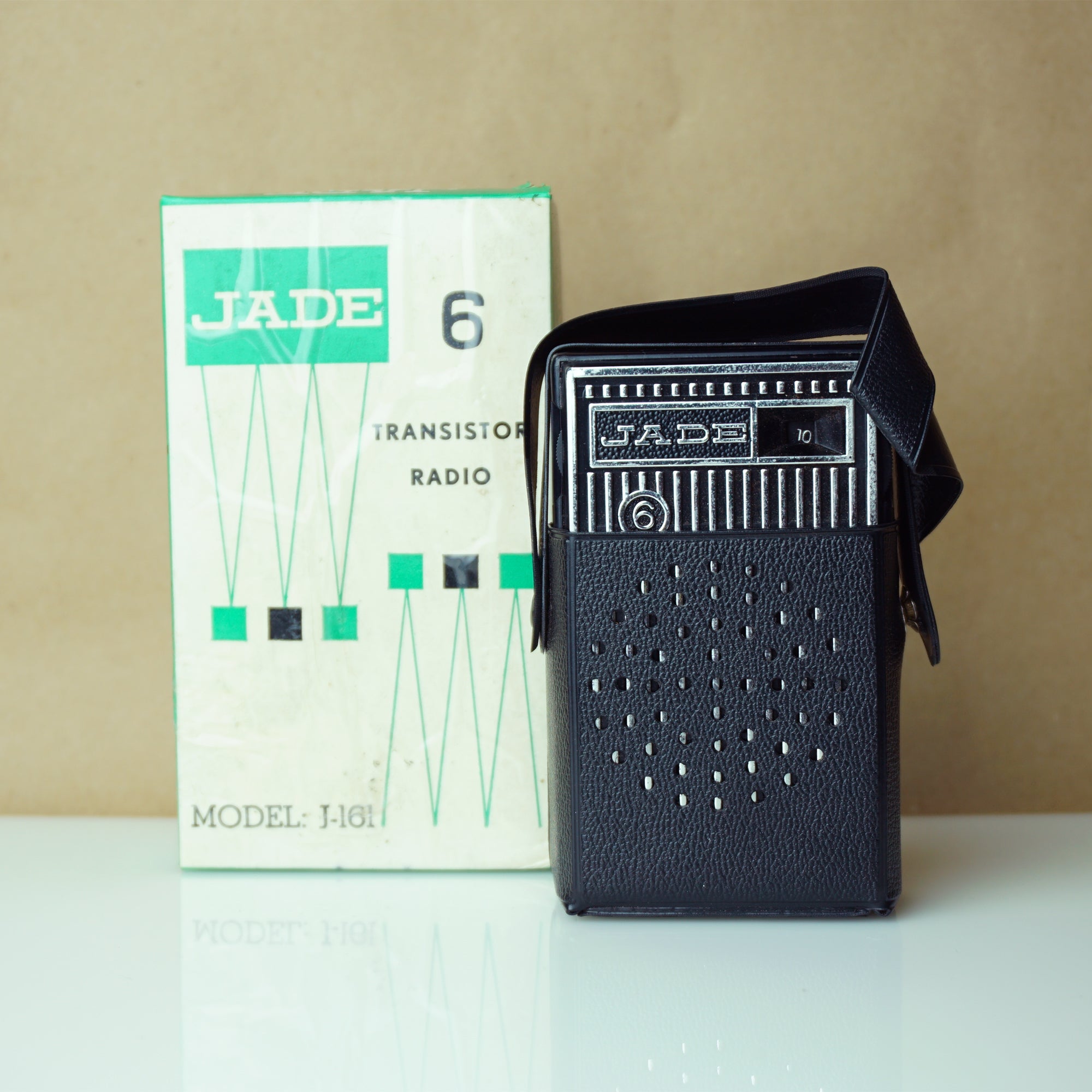This is a photograph capturing a vintage handheld transistor radio and its original packaging. The radio, positioned on the right, is a compact, black device designed to fit nicely in a shirt pocket, and it's housed in a semi-leather carrying case complete with a strap for easy portability. The front of the radio features a simple design with a speaker, made up of a series of small holes, and the name "JADE" emblazoned on it in silver text. A small display likely indicates the current radio channel, and the model number "6" is also visible. To the left of the radio stands its white box, adorned with colored squares and the "JADE" branding in white text over a green rectangle. The box, labeled as a "6 transistor radio" and identified with the model number "J16T," mirrors the streamline simplicity of the radio itself, offering a nostalgic glimpse into past audio technology on a white countertop backdrop with a subtle brown paper background.